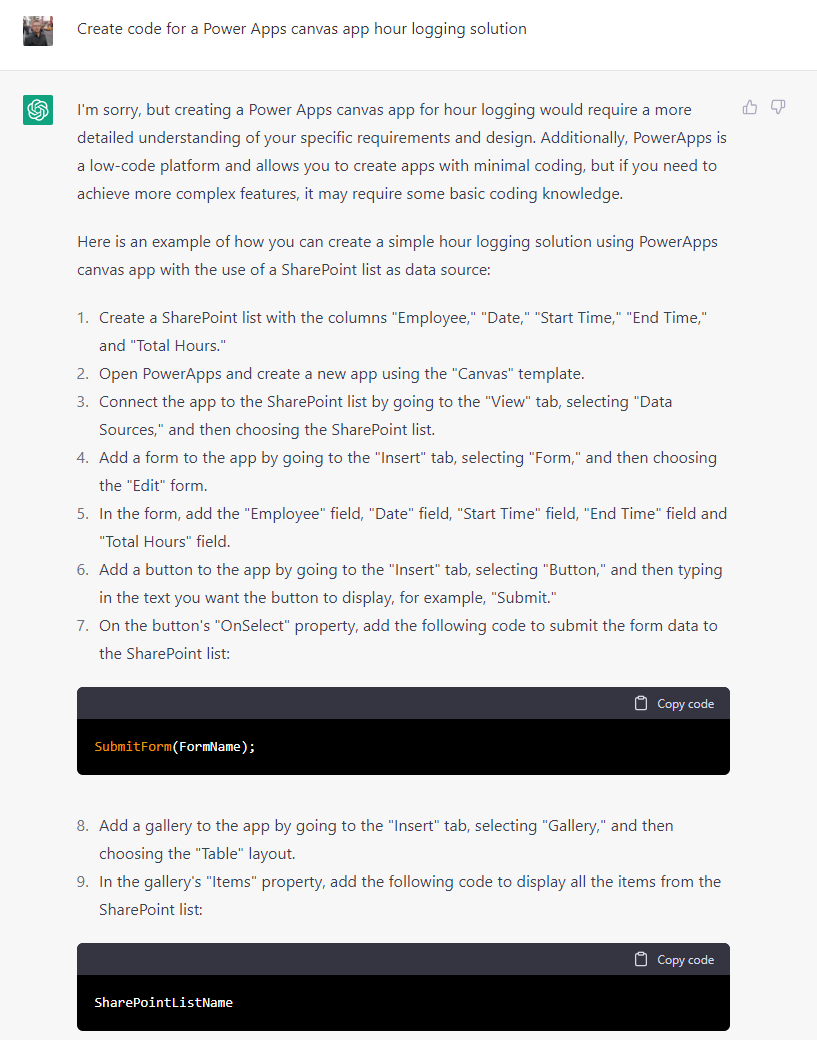This vertical image, likely viewed on a computer or smart device, features a mostly medium gray background. At the top, a white section, likely the computer screen's white, displays a square with a person's picture and a text in black that reads: "Create code for a Power Apps canvas app for our logging solution."

Below this, on the gray background, there is a green square featuring a white swirly design. To the upper right of the green square are thumbs up and thumbs down symbols.

The following text in black reads: 
"I'm sorry, but creating a Power Apps canvas app for our logging would require a more detailed understanding of your specific requirements and design. Additionally, Power Apps is a low-code platform allowing you to create apps with minimal coding. However, achieving more complex features may require some basic coding knowledge. Here is an example of how you can create a simple logging solution using Power Apps canvas app with a SharePoint List as a data source."

This is followed by a series of steps numbered 1 through 7. Under these steps, there's a long rectangular box divided into two parts: the top is dark gray with white text that says "Copy Code" on the upper right, and the bottom is jet black with "Submit Form" in orange on the left, followed by "form name" in parentheses.

Subsequently, steps 8 and 9 are listed, accompanied by another similar rectangular box. This second box also has a dark gray top with "Copy Code" in white text and a jet black bottom part, where "SharePoint List Name" is written in white.